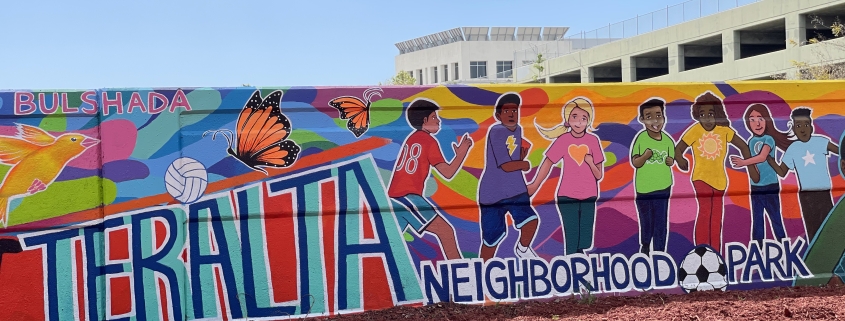In this vibrant mural painted on a wall in a park, the upper left section displays the word "Bullshotta" in pink. Just below this, a vivid yellow bird perches on a green branch. Prominently spread across the mural in striking blue letters with a red background is the word "Teralta," decorated with a white soccer ball perched atop the letter 'A'. The lower part of the wall reads "Neighborhood Park" in blue letters outlined in white, with another soccer ball nestled amongst the words. The scene is sprinkled with a multitude of colorful elements, including a monarch butterfly and various children engaged in soccer. Among these children, a little girl in a soccer jersey stands out, accompanied by a lady in a pink shirt and blue jeans with blonde hair. There are also a young boy in a green shirt and blue jeans with black hair, a black girl sporting a yellow shirt and red jeans with long hair, a white girl with long brown hair in a blue shirt and blue jeans, and a black boy with short black hair wearing a blue shirt and brown jeans. The engaging tableau is set against a backdrop that includes a portion of a cream-colored building, a light powder blue skyline, and a glimpse of a white stucco parking garage with a solid painted fence underneath. The mural, filled with ethnic diversity and vibrant colors, also features various butterflies and birds, encapsulating a lively neighborhood scene with enthusiastic children from different cultures playing soccer amidst the brown mulch spread in front of the wall.